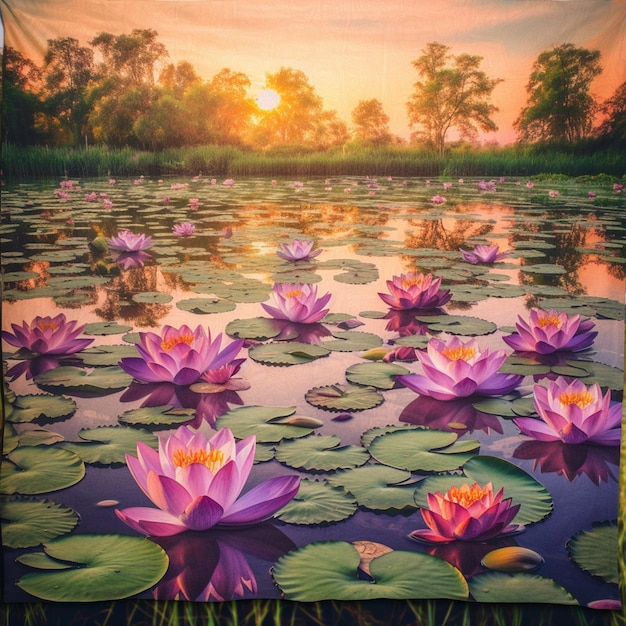This detailed image captures an extraordinarily realistic drawing of a vast lily pond during sunset, possibly displayed on a large banner-like cloth. The pond is richly adorned with lily pads and striking purple lilies with vivid yellow centers, creating an enchanting, dreamy ambiance. The water's surface is incredibly still, colored in a deep, dark blue that seamlessly reflects the golden peach sky, casting a warm hue over the scene. Surrounding the pond in the background, tall green grasses reminiscent of a marshland frame the view, while large green trees stand majestically under the sunset. The lower edge of the image reveals actual grass, blending the outdoors with the artwork, adding to the immersive, tranquil atmosphere.